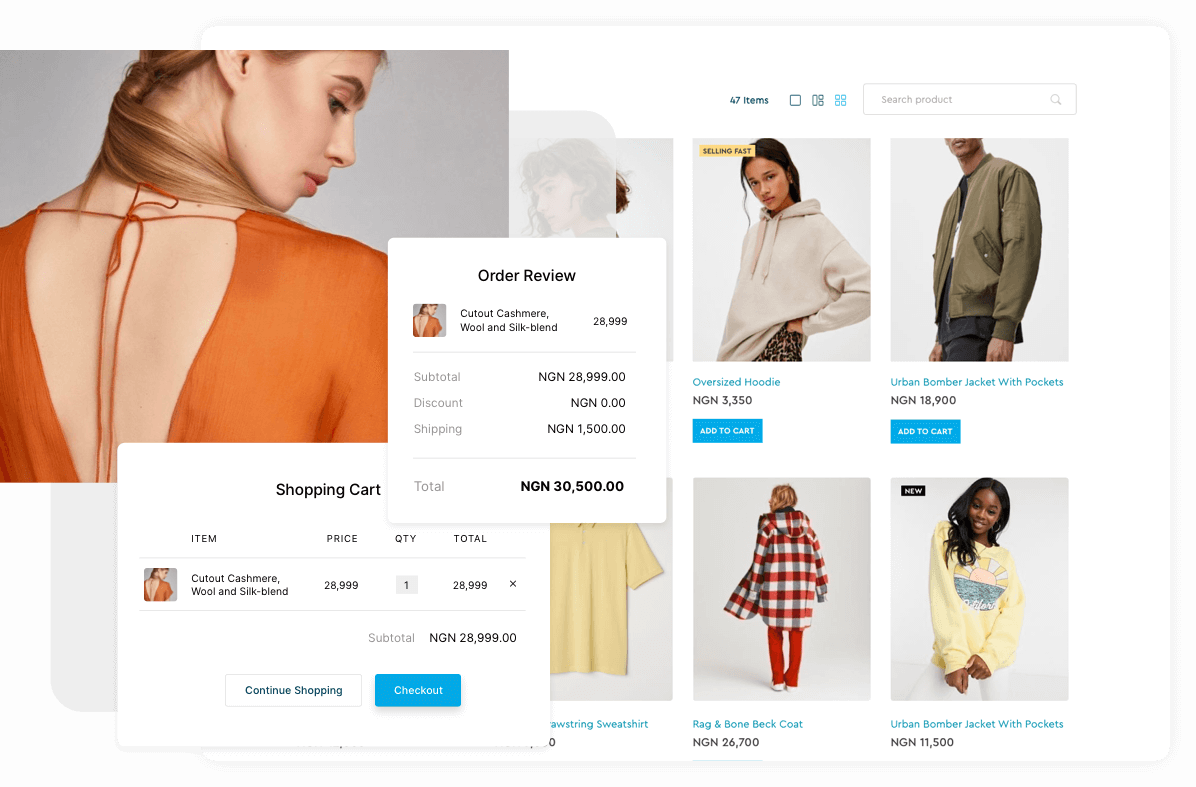This screenshot captures a detailed view from a website, showcasing a variety of visual elements and individuals. On the left side of the image, a large square with a gray background prominently displays the back of a woman. She is dressed in an open-back gray shirt or dress, with a delicate gray string securing it at her shoulders and trailing down her exposed back. Her brownish blonde hair is styled in a ponytail, cascading down her neck and draping over her shoulder in front. Her head is turned to the right, revealing the right side of her face, including her eye, nose, mouth, and part of her right ear. She has fair skin.

Adjacent to this image on the right, there is a faded picture depicting a girl with curly hair facing left. Beside her, another woman, who has darker skin and black hair, is shown in a gray hoodie with her arm positioned on her waist. This image is cropped at her waist. Additionally, a man in a green jacket is visible, facing left with his hands down at his sides. This image cuts off just below his hands, only revealing the top of his mouth. He also has darker skin.

Beneath these images, there is blue and black text accompanied by a blue button with white text. Another image below the man shows a very dark-skinned woman with black hair, smiling directly at the camera. Her hands are clasped together, and she wears a loose yellow sweatshirt. This image is cropped at her waist.

To her left, a woman with her back to us is seen wearing a long white and red checkered jacket paired with solid red pants. Her hair color is indistinct. Next to her, a plain yellow t-shirt is partially obscured by two pop-ups. One pop-up, titled "Shopping Cart," contains an icon image, text, and a blue button with white text. Above it, another pop-up titled "Order Review" displays similar information along with a price.